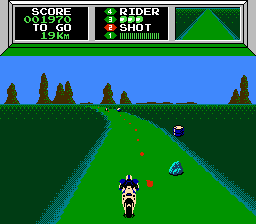This image is a highly pixelated, vintage-style video game screenshot reminiscent of the Game Boy era, characterized by its small, square format. Dominating the scene is a bright green road that stretches from the foreground to the horizon, curving to the left. A motorcycle, positioned center-frame, is prominently moving forward on this road. On the road's right-hand lane, a rock obstacle is visible, while the center lane is marked by small red lines. In the distance, near the horizon, two more motorcyclists can be discerned, adding to the sense of depth and perspective. Additionally, a person stands on the side of the road to the immediate right of the center lane.

The upper portion of the image features an information display panel with a retro aesthetic, using white, green, and red colors. This panel provides crucial gameplay details, such as the current score, the player's rider, available shots, and other metrics. To the right of this HUD (Heads-Up Display) panel, there is a detailed close-up of the road itself, rendered in greens, blues, and reds, further emphasizing the game's vintage charm.